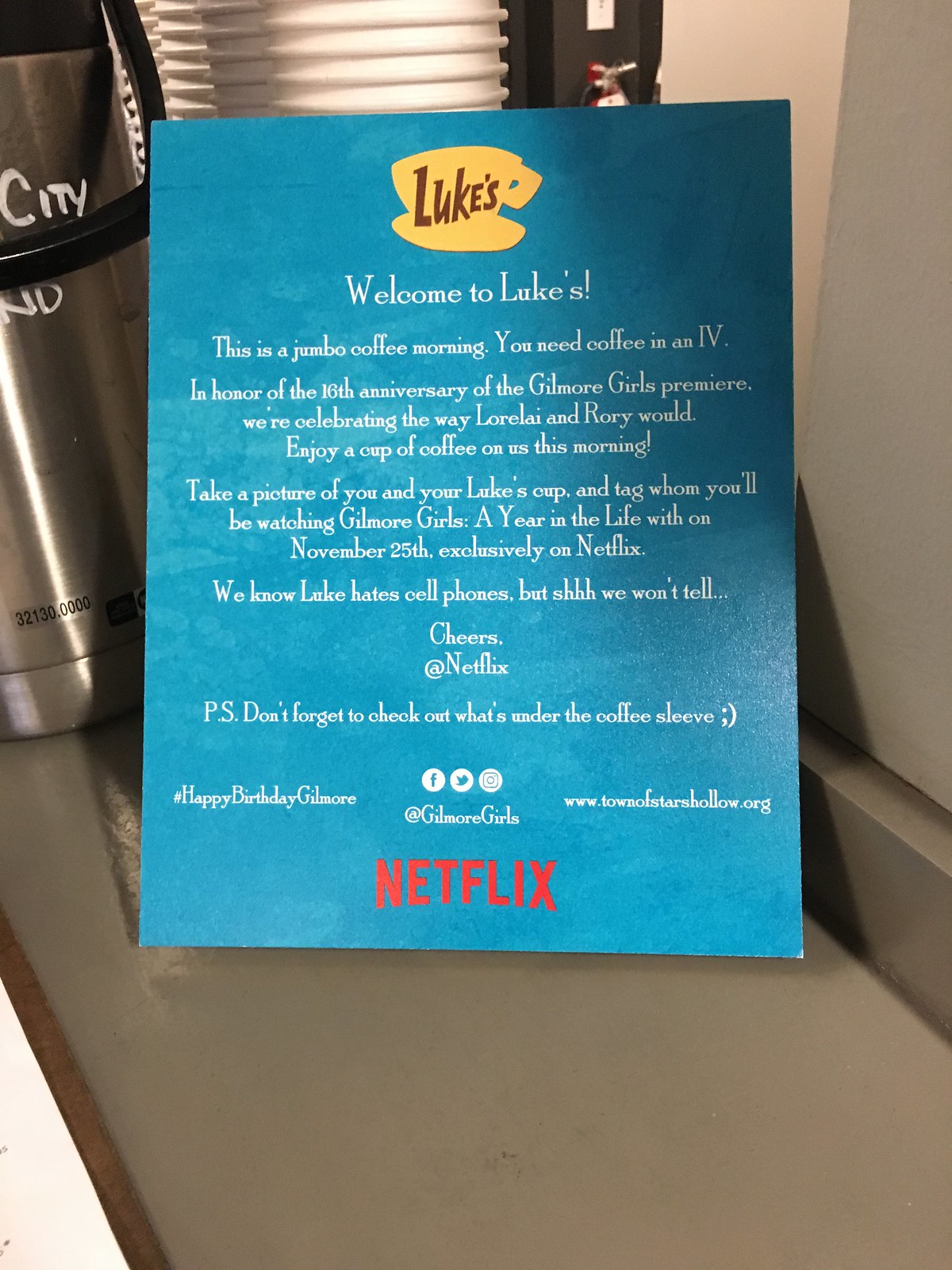The photo features a detailed sign on a small table next to a stack of paper coffee cups and a silver coffee urn. The sign, set against a dark gray background and possibly placed inside some sort of dining or gathering area, announces: "Welcome to Luke's." At the top of the sign, there is a yellow coffee cup with "Luke's" printed in brown. The text reads: "This is a jumbo coffee morning. You need coffee and an IV. In honor of the 16th anniversary of Gilmore Girls premiere, we're celebrating the way Lorelei and Rory would. Enjoy a cup of coffee on us this morning. Take a picture of you and your Luke's cup and tag whom you'll be watching Gilmore Girls: A Year in the Life with on November 25th, exclusively on Netflix. We know Luke hates cell phones, but shh, we won't tell. Cheers! - Netflix." At the bottom of the sign, there is a red Netflix logo with social media icons and the handle @GilmoreGirls. The scene is devoid of people, focusing solely on the celebratory setup aimed at fans of the iconic TV show.